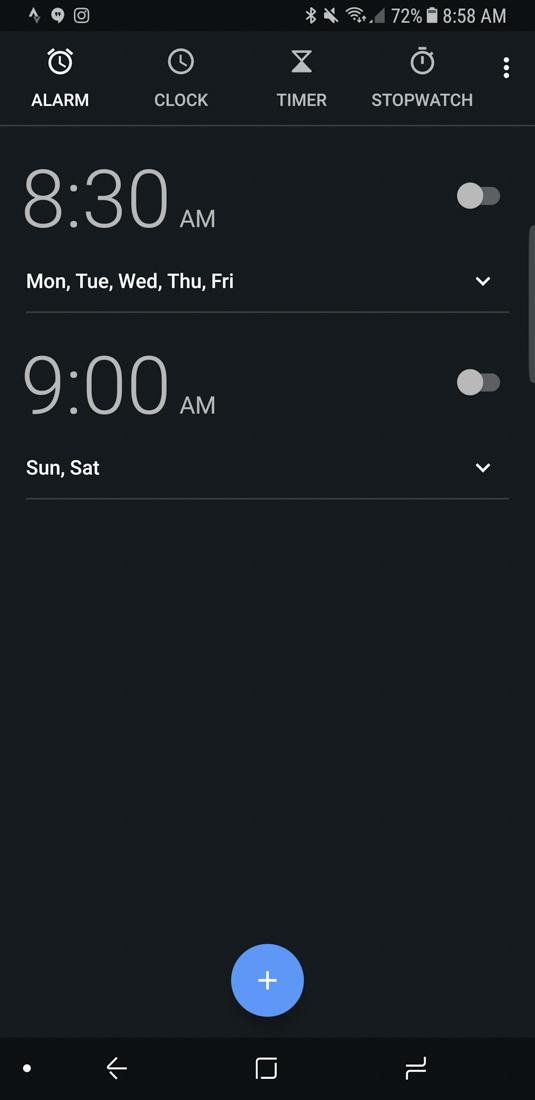This screenshot shows the alarm setting interface on a smartphone. The background is entirely black. In the upper right-hand corner, the time is displayed as 8:58 a.m., with the battery life at 72% and the sound muted. At the top of the screen, there is a white alarm clock icon labeled "Alarm." Below this are three gray icons with their respective labels: "Clock," "Timer," and "Stopwatch."

The alarm settings are prominently displayed below these icons. The first alarm is set for 8:30 a.m., with the days Monday, Tuesday, Wednesday, Thursday, and Friday listed underneath it. To the right of this alarm is a toggle button. The second alarm is set for 9:00 a.m., with the days Sunday and Saturday listed underneath, and another toggle button to the right. Each section is divided by thin, very light gray lines, providing a clear separation between different elements.

At the bottom of the screen, there is a blue circle with a white plus sign in the center, suggesting the option to add a new alarm. This detailed layout clearly indicates that this is a screenshot of the alarm setting feature on a smartphone.